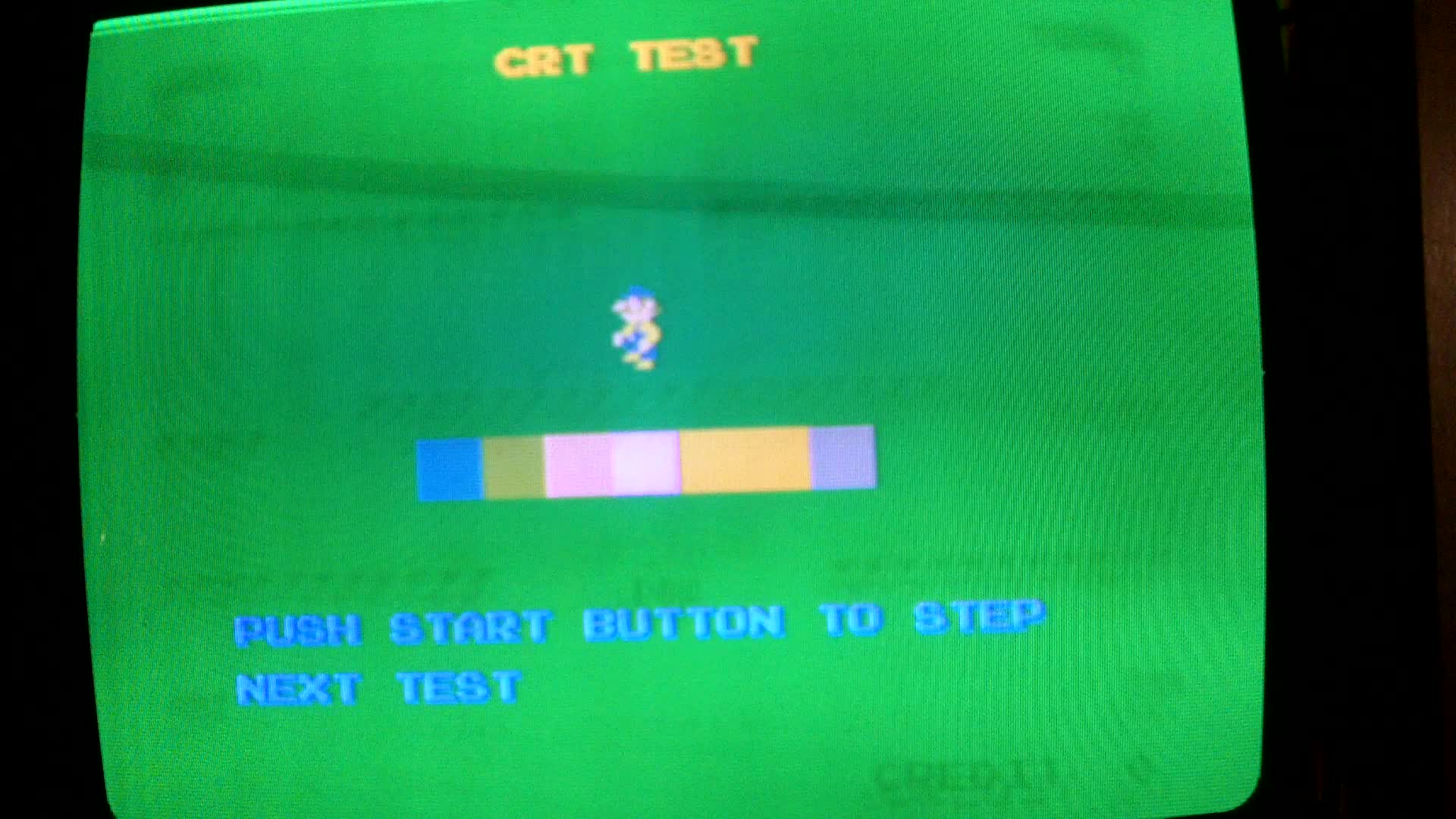This is a detailed caption for the photo:

"The image depicts a television screen displaying what appears to be a video game or instructional test interface. At the top, the screen prominently features the text 'CRT Test' in yellow. Below this, there is an icon resembling a small person next to a larger person. The central part of the screen showcases a gradient color scheme transitioning from blue to a pinkish hue. Beneath this gradient, the instructions 'Push start button to step' are displayed, followed by 'Next test' in smaller lettering. The entire screen has a lime green background, with visible scan lines characteristic of CRT displays. In the bottom right corner, the text 'Credit 0' is visible, indicating the video game nature of the screen."